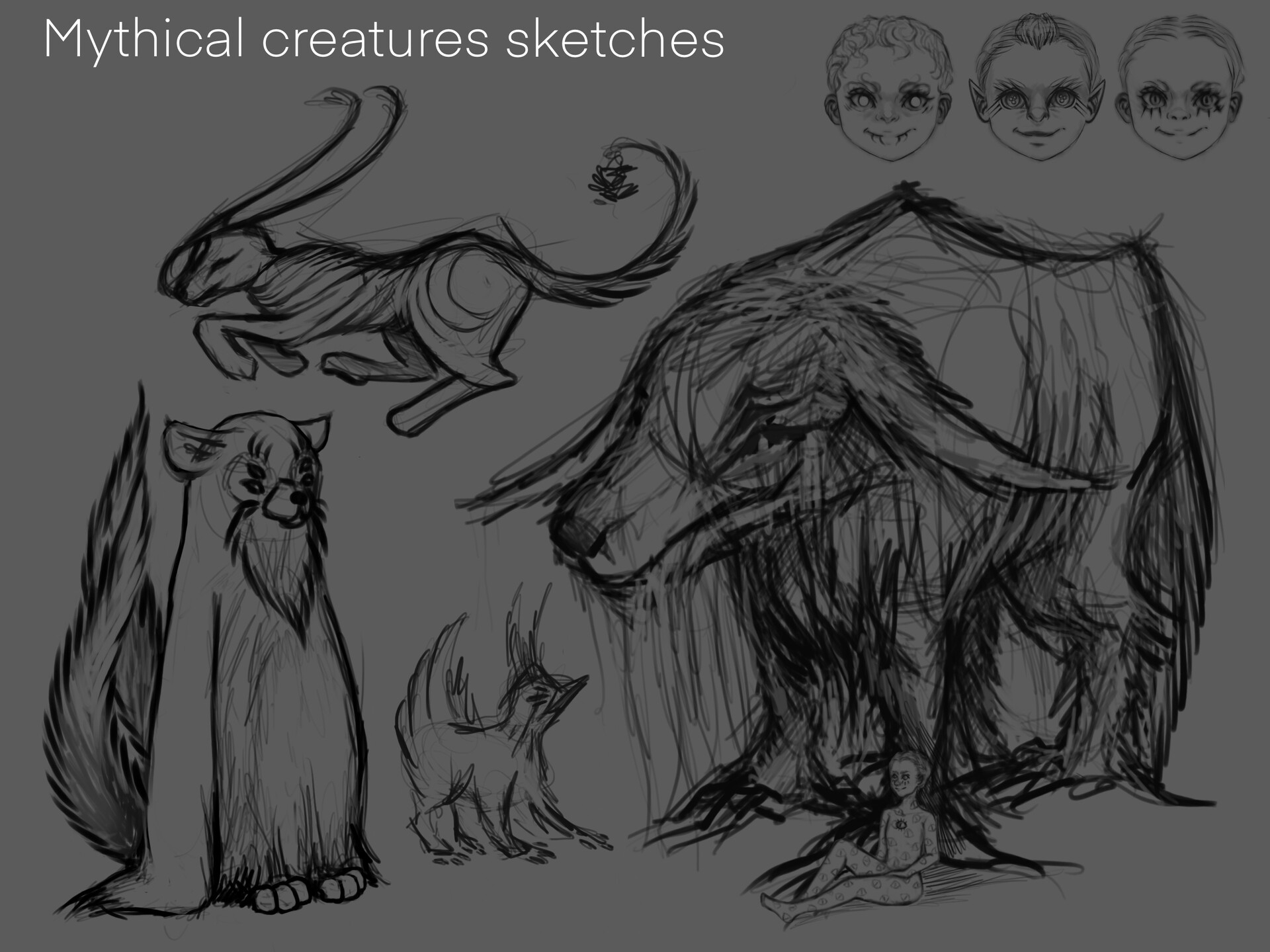The grayscale image, captioned "Mythical Creature Sketches" in white sans-serif font at the top left, showcases various meticulously detailed sketches of mythical creatures on a gray background. On the top right, three sinister children's faces hover with unsettling, exaggerated features like vacant, pupil-less eyes, sinister smiles, and peculiar ears, giving them a devilish appearance.

In the bottom left corner, a fluffy, bipedal creature with fox-like ears, a goat-like beard, and four eyes stands with penguin-like flippers and intertwined tails. Its body exudes a mix of bear and fox elements.

Next to it is a dog-bird hybrid resembling a small, lively terrier with tall, erect ears and a beak, paired with a duck-like tail, imbued with an animated, excited posture.

Dominating the right side is a colossal beast, blending the traits of a dog and a cow, with a Labrador-esque face and a shaggy, bovine body. It towers over a small, reclining figure leaning against its paw, emphasizing its immense size.

Nearby, in the upper left section below the caption, a feline-deer hybrid in mid-motion features a cat-like body, a long tail with a flower at its tip, and delicate whisker-like antlers arching over its form.

Completing the surreal tableau are various other smaller sketch creatures scattered around, each blending characteristics of familiar animals into fantastical new forms, enhancing the enchanting and eerie quality of the artwork.